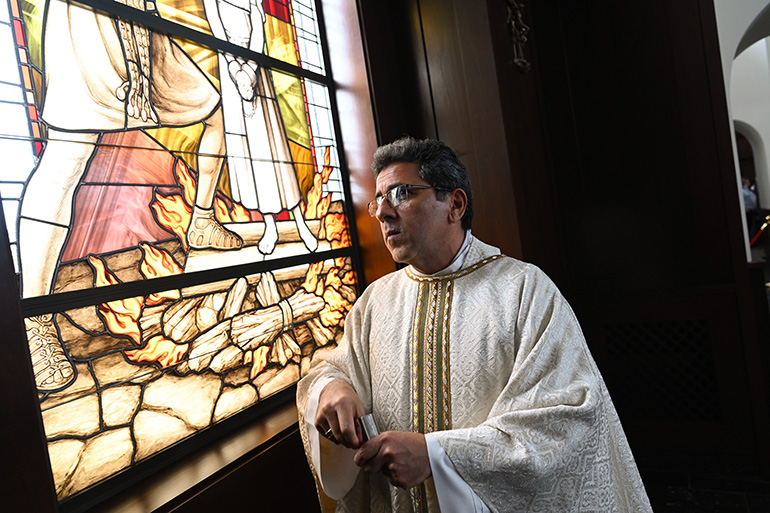The photograph captures a Roman Catholic priest in his 40s, with dark hair, wire-rimmed glasses, and brown skin, standing thoughtfully inside a church. The priest, adorned in white vestments with intricate gold and green trim down the front, holds a small Bible in one hand. He leans contemplatively against a wall, gazing out of a stained-glass window beside him. The window artwork, partially visible, dramatically depicts St. Joan of Arc being burned at the stake, with logs and flames at her feet, and a soldier in sandals and a skirt leaning towards the saint, whose hands are chained. The scene is set within a church interior featuring dark wood paneling on the right side of the image, emphasizing a realistic and representational artistic style.